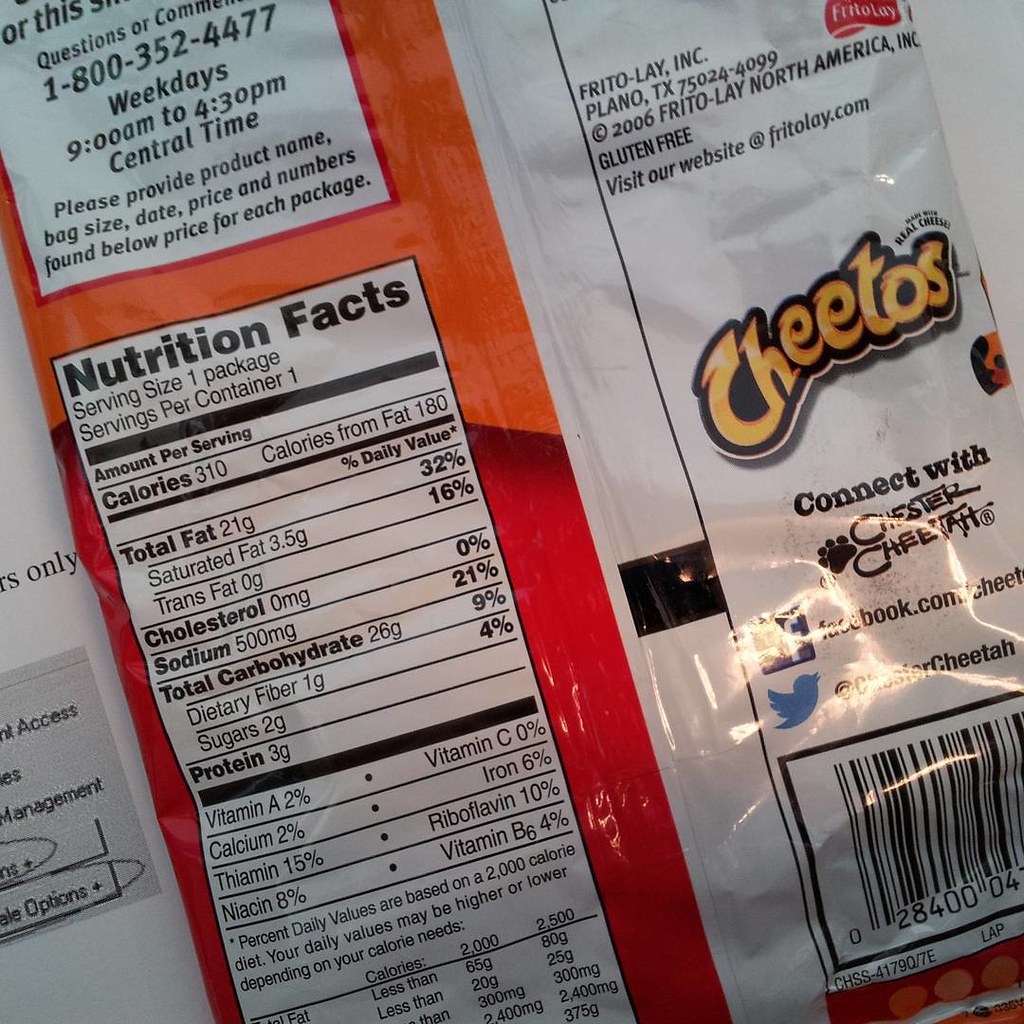This image features the back of a Cheetos package, made from thin plastic with a predominantly orange and red color scheme. The back label is divided into three white panels, each providing different information. The first panel displays the Nutrition Facts, including details such as 310 calories, 21 grams of total fat, and 0 milligrams of cholesterol. The second panel offers customer service information, including contact details for questions or comments. The third panel contains company information and the UPC code. Additionally, it invites consumers to connect with Chester Cheetah on Facebook and Twitter, enhancing brand engagement through social media platforms.